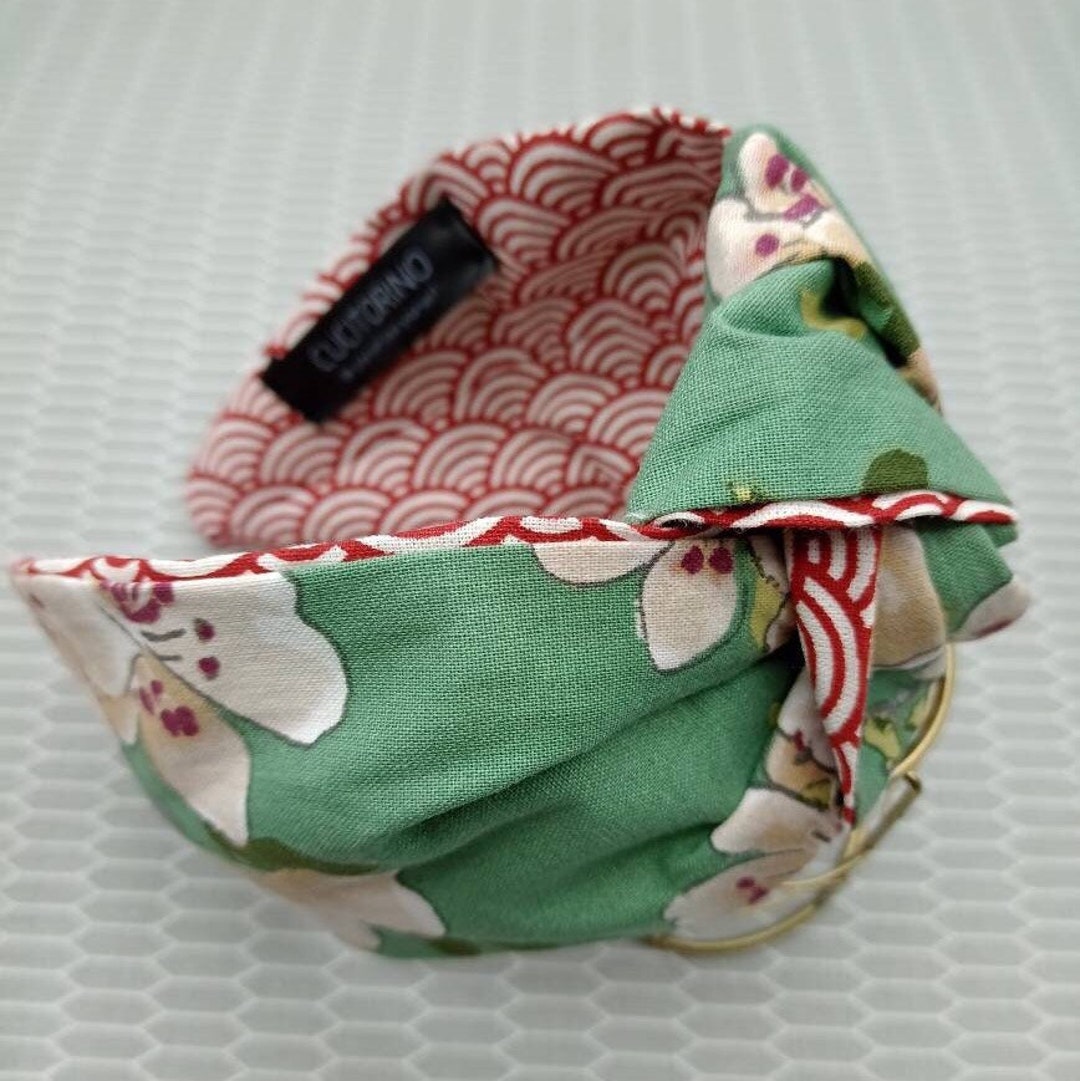This image features a folded fabric object, possibly a hat, bib, napkin, or towel, placed against a variegated gray and white background that resembles a tablecloth. The background has a pattern of gray hexagons and white outlines creating a solid and consistent design throughout. The fabric itself presents a two-toned aesthetic: the outer layer is a light sage green adorned with delicate white flowers, some showcasing pink stamens and purple dots, while the inner layer displays a red and white fan-shaped pattern with curved lines and semi-circles.

A black label inside the fabric bears the text "C-U-C-I-T-O-R-N-O," though the smaller text beneath is illegible due to image blurriness. Additionally, the way the fabric is folded reveals the contrasting inner and outer patterns, making it challenging to identify its exact purpose. Notably, the fabric features brass braces at the bottom section, which contribute to the twisted and enigmatic appearance of the item.